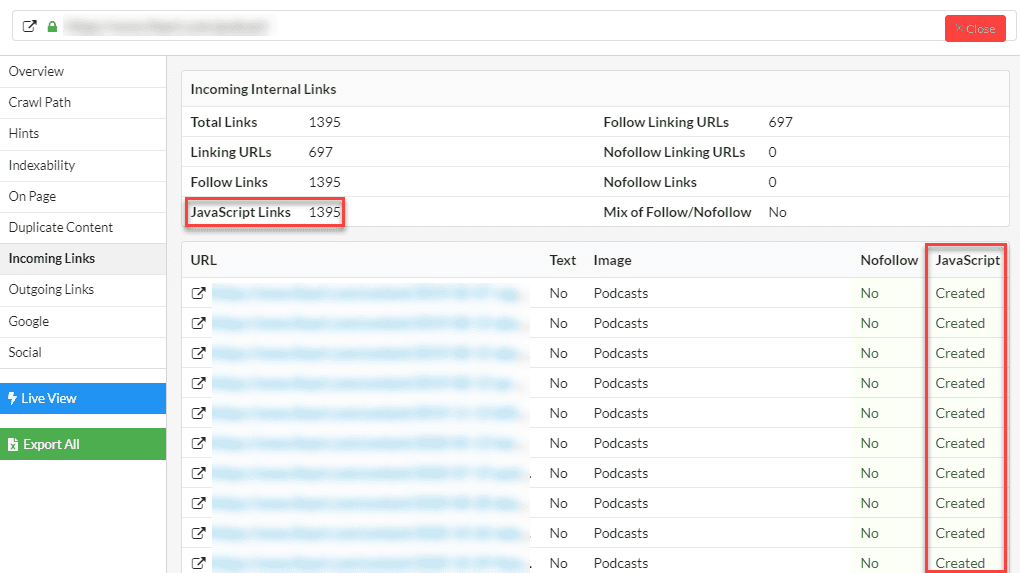This screenshot captures a detailed view of a website's analytics page, focusing on internal linking data. The interface is divided into two primary sections: a vertical menu on the left and a detailed content analysis area on the right.

**Left Menu:**
The vertical menu occupies the left-hand side, featuring several navigational options:
- **Overview**
- **Crawl Path**
- **Hints**
- **Indexability**
- **On Page**
- **Duplicate Content**
- **Incoming Links** (highlighted in grey to indicate it is the current selection)
- **Outgoing Links**
- **Google**
- **Social**

Below these options, there are two colored buttons:
- **Live View**: Positioned in a blue box with a lightning bolt icon.
- **Export All**: Located in a green box with a spreadsheet icon.

**Main Content Analysis Area:**
This section is divided into two segments:

1. **Incoming Internal Links:**
   - **Column Headings and Data:**
     - **Total Links:** 1,395
     - **Linking URLs:** 697
     - **Follow Links:** 1,395
     - **JavaScript Links:** 1,395 (highlighted with a red box)
     - **Follow Linking URLs:** 697
     - **No Follow Linking URLs:** 0
     - **No Follow Links:** 0
     - **Mix of Follow/No Follow:** No

2. **URLs List:**
   - This section contains around 10 blurred URLs, each on separate rows with the following columns:
     - **Text:** All entries say "No"
     - **Image:** All entries say "Podcasts"
     - **No Follow:** All entries say "No"
     - **JavaScript:** All entries say "Created" (highlighted with a red box)

This screenshot provides a comprehensive view of the website’s internal link structure, emphasizing the prevalence of JavaScript links and the categorization of various links and URLs.